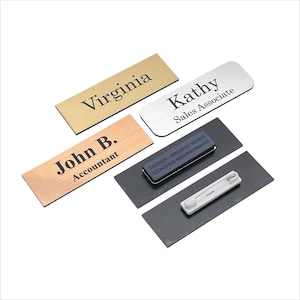The image displays a collection of nameplates arranged neatly against a wood background, forming a triangular pattern. At the top, there is a gold nameplate reading "Virginia" in black letters. Just below this, to the left, is a brass-colored nameplate with "John B." in bold black text and "Accountant" beneath in smaller black font. To the right of John B.'s nameplate is a rectangular, silver nameplate with rounded edges, displaying the name "Kathy" in large black font and "Sales Associate" below in a smaller font. Below these three nameplates are two additional nameplates flipped upside down, showing their backs. One of these has a blue magnetic attachment with the partially legible warning "caution," and the other has a pin attachment, meant for securing through fabric.